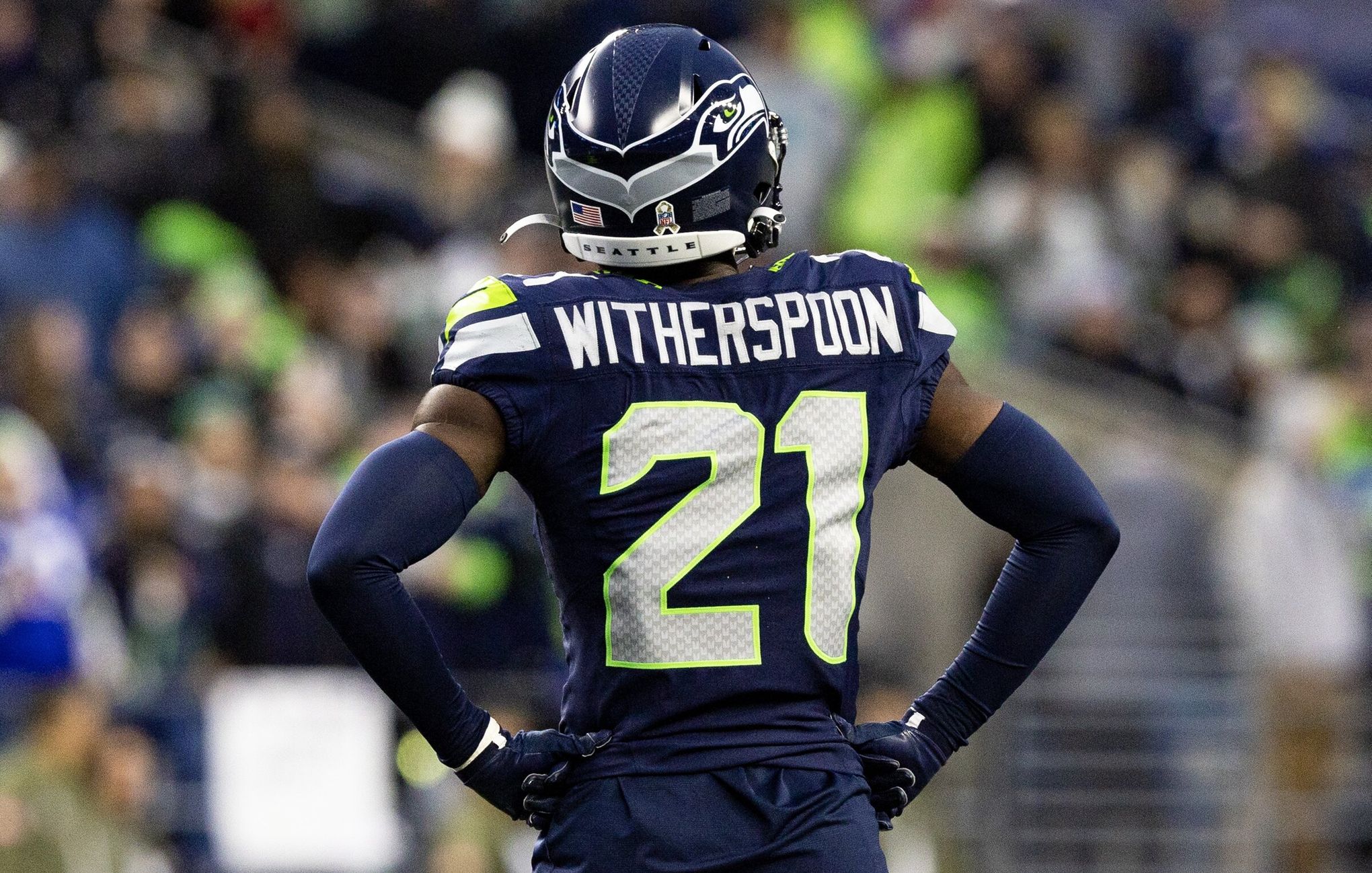This photograph showcases a dark-skinned American football player from behind, revealing a wealth of detail on his uniform and stance. He dons a navy blue jersey, pants, and long sleeves that extend from his wrists to beneath his biceps, along with matching blue gloves. His arms are bent at the elbows, with his hands resting on his hips and his thumbs positioned on his lower back. His navy blue helmet features the Seattle Seahawks emblem: a blue and gray bird with a white beak and a striking bright green eye, alongside an American flag emblem and a golden ribbon logo with an NFL shield. The word "Seattle" is inscribed in black text at the bottom of the helmet. 

The back of his jersey prominently displays his name, Witherspoon, in large white letters, above the number 21. The number is gray, outlined in neon green, and spans the majority of his back. Each shoulder of his jersey is adorned with a green and white stripe. 

In the blurred background of the image, hints of a crowd and stadium stairs can be discerned, with occasional bright neon yellow-green spots standing out, possibly from fans' clothing or lights. The focus on the player's detailed uniform and dynamic pose contrasts sharply with the indistinct, yet bustling, scene behind him.